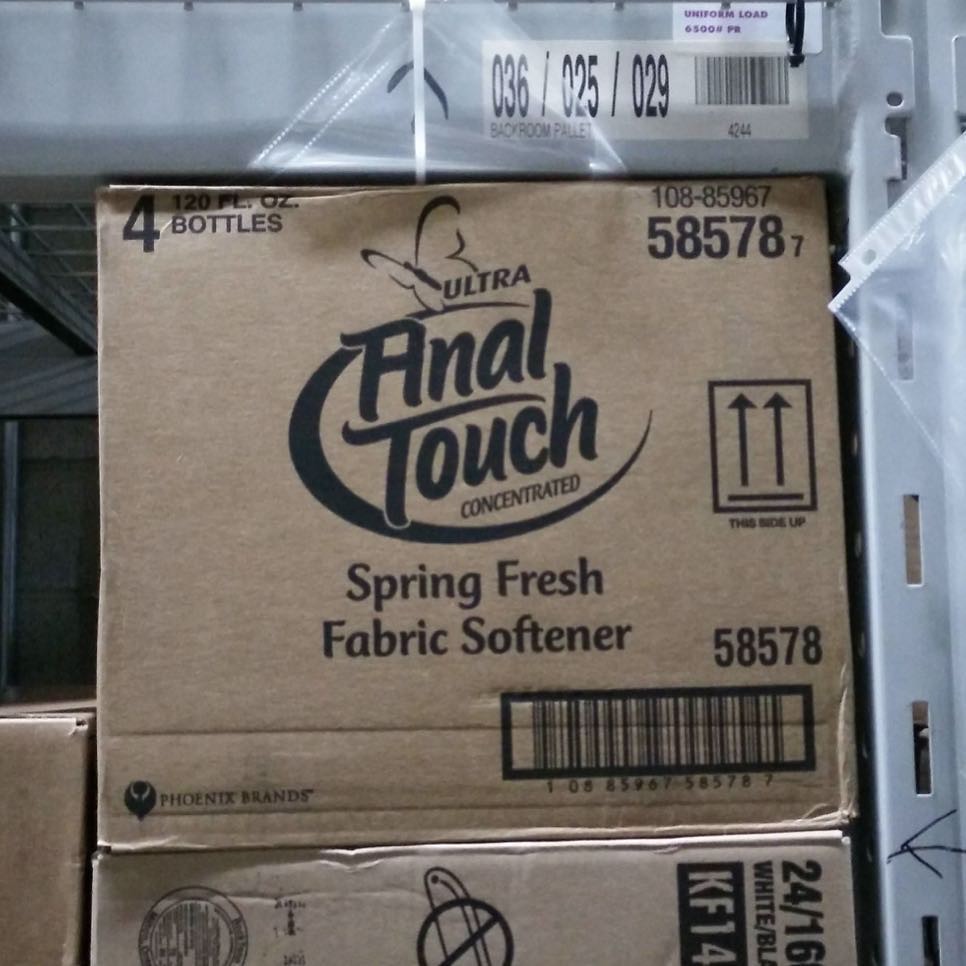The image depicts a storage area, likely within a company or factory, showcasing cardboard boxes and metal shelving units. Central to the frame is a brown box with black text, prominently displaying "Ultra Final Touch Concentrated Spring-Fresh Fabric Softener." The box also includes several other details: a bold "This Side Up" warning, Phoenix Brands labeling, and multiple product codes such as "58578" and "108-85-96-7." Notably, a sticker reads "Uniform Load" in purple and specifies that the box is intended for "120 fluid ounce bottles." 

In addition to the central box, there is a partial outline of another box below it and the bottom left corner features a cutoff view of a third box. The metal shelving, described as gray with rectangular slits, appears to house the boxes, with vertical rods visible on the far right and top of the image. The overall scene evokes a utilitarian storage unit atmosphere, indicative of a back-room or warehouse setting.